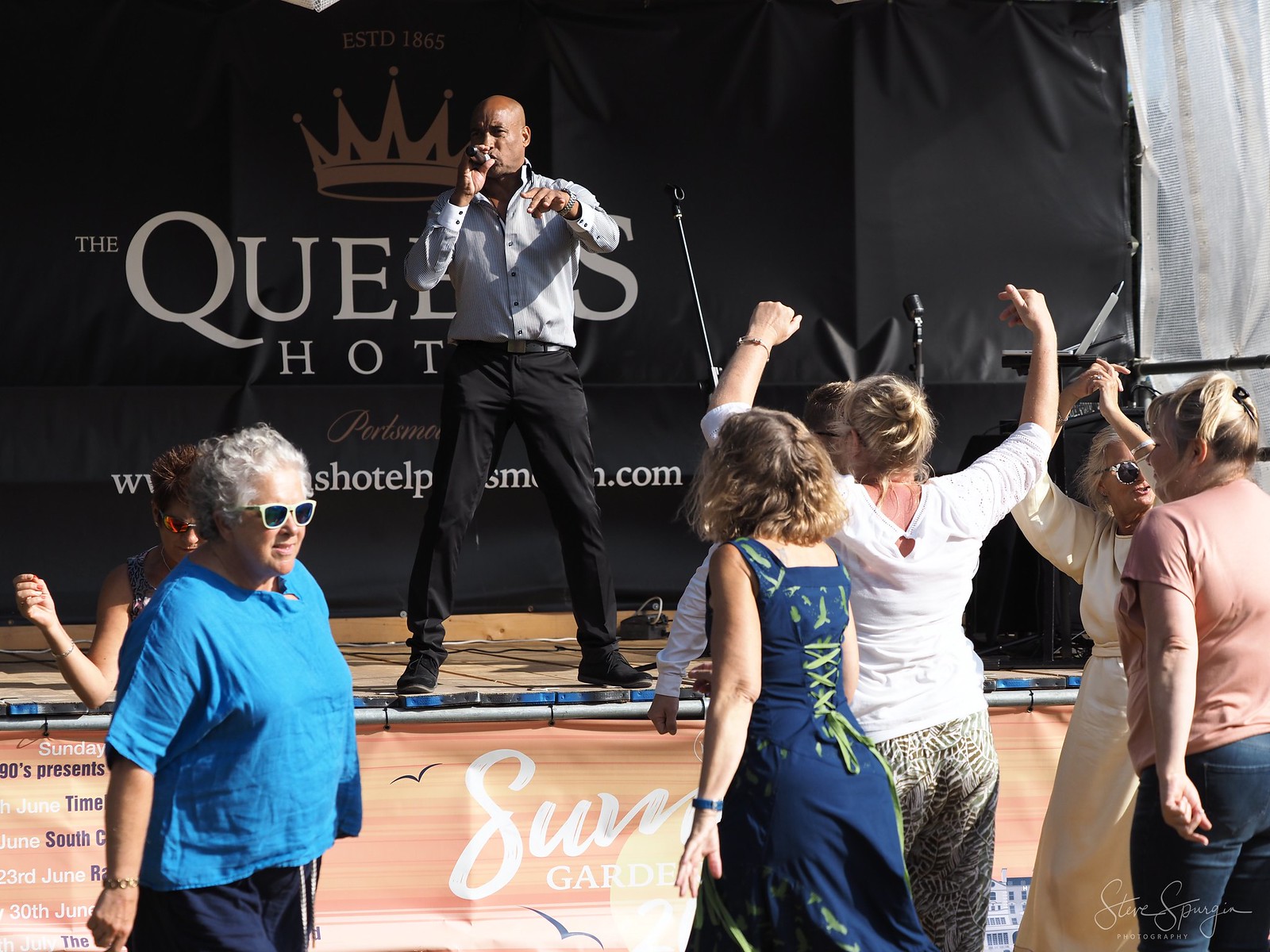In a vibrant outdoor concert scene, a well-dressed African American man commands the stage, singing passionately with a cordless microphone in hand. Clad in crisp black slacks and a light-colored long-sleeved button-down shirt, the bald performer stands confidently under a black banner that reads "The Queen's Hotel." Some faint words, including a .com address, peek through the lively background but are mostly obscured. Below the stage, a pink banner inscribed with "Sun Gardens" adds a splash of color. In front of the stage, a group of older white women joyfully dances. Their attire ranges from casual t-shirts and slacks to longer, more flowing dresses, and some wear sunglasses, indicating the event's outdoor setting. The lower right corner of the image bears a photographer's partially visible signature, possibly "Steve" followed by an unreadable surname. The joyful atmosphere captures a moment of shared enjoyment and vibrant music.